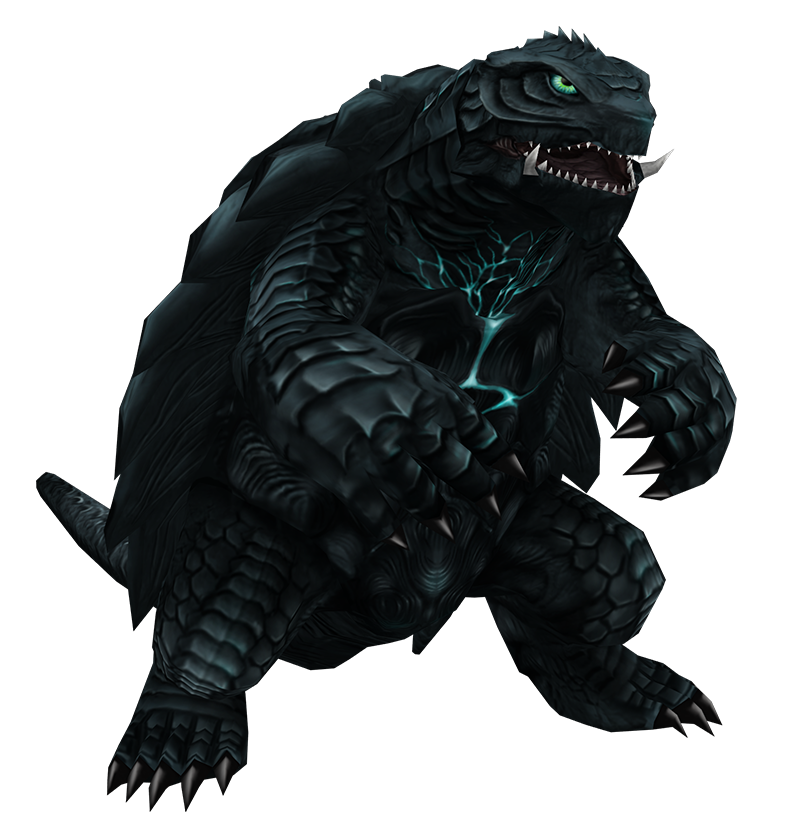The image is a highly detailed, computer-generated 3D rendering of a monstrous, bipedal turtle-like creature set against a stark, all-white background that gives the impression of it floating in a white void. The square composition of the image makes for a symmetrical view of the creature. This kaiju-like monster stands upright on its hind legs with its front limbs extended forward, each ending in sharp, slightly bent claws. The dark, grayish-black scales covering its body contrast vividly against the white backdrop. It possesses a large, ridged shell on its back, typical of a traditional turtle, though more menacing in appearance. From its back protrudes a tail that stretches slightly towards the top right and left corners of the frame. The creature's fearsome visage includes glowing green eyes and an open mouth displaying several sharp teeth and two pronounced lower fangs, alluding to its aggressive nature. A distinctive glowing blue line runs vertically along its stomach, adding to its otherworldly aesthetic.